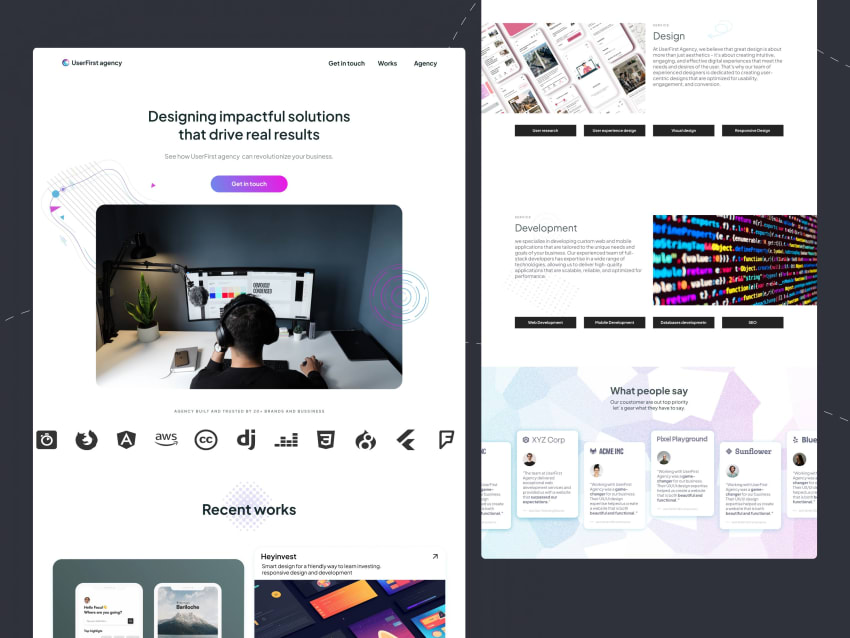A captivating homepage of the "User-First Agency" greets visitors with a striking tagline in bold letters: "Designing impactful solutions that drive real results." Positioned in the top left corner, the agency's title is prominently displayed, while the top right corner invites engagement with the prompt, "Get in Touch."

At the center of the page, a compelling call-to-action reads, "See how User-First Agency can revolutionize your business." Below this, a stylish "Get in Touch" button stands out with its purple background and white lettering, inviting further interaction.

Beneath this primary section, an image captures a man engrossed in work at his computer, donning headphones and a microphone, symbolizing a modern, professional environment. This is followed by a showcase of esteemed partners, including recognizable names like Amazon and Fandango, among others.

The page is organized into a well-structured layout, split between informative sections on the left and right. On the left, under the headline "Design," a brief paragraph introduces the agency's approach to design, accompanied by various tabs for deeper exploration. Below, another section labeled "Development" follows the same format, with a descriptive paragraph and navigable tabs.

Finally, the bottom section features testimonials under the heading "What People Say," providing reviews from satisfied clients to bolster the agency's credibility and success.

This meticulously arranged homepage offers a comprehensive overview of the User-First Agency's mission, services, and reputation, effectively engaging potential clients with its clean, professional design and user-friendly interface.